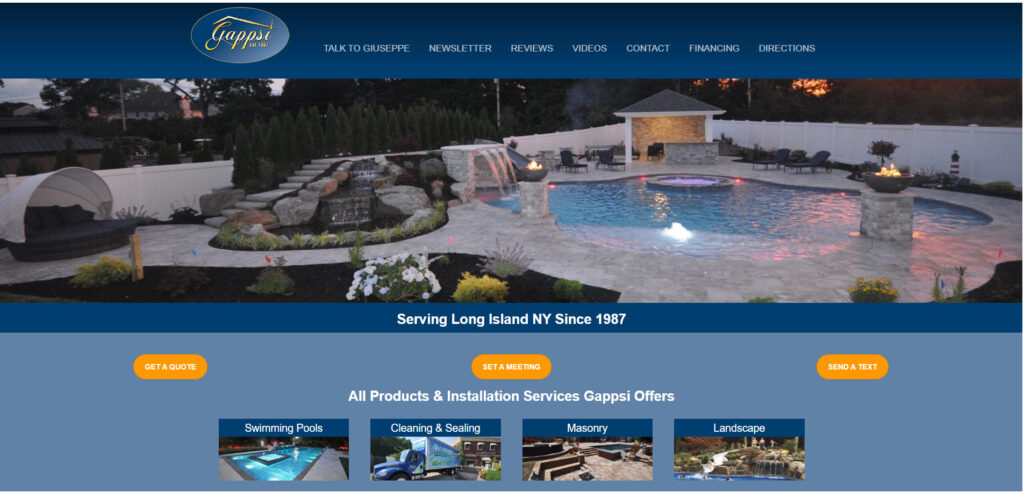The webpage for Gapsi, a company specializing in building work and garden maintenance, features a rich blue color scheme. At the very top, there is a full-width dark blue bar with the company's oval logo prominently displayed. The logo features the name "Gapsi" in yellow cursive handwriting, accentuated by a small roof-like inverted 'V'. The navigation menu, also in white text, includes options such as "Talk to Giuseppe," "Newsletter," "Reviews," "Videos," "Contact," "Financing," and "Directions."

Below the navigation bar, a full-width photograph showcases an ornate swimming pool. Though slightly low resolution, the image captures the pool's irregular, oval shape surrounded by concrete slabs. The scene is enhanced by outdoor fire pits on plinths and a small hut at the back, possibly for barbecues or as a sweat hut. On the left side of the pool, steps lead up to an upper level that features a waterfall-like structure.

A narrow dark blue band beneath the photograph states, "Serving Long Island NY since 1987." Just below, on a slightly lighter blue background, are three orange oval buttons labeled "Get a Quote," "Set a Meeting," and "Send a Text." Further down, a section details the products and installation services offered by Gapsi: Swimming Pools, Cleaning and Sealing, Masonry, and Landscape. Each service is accompanied by a small illustrative picture, providing clickable options for visitors.